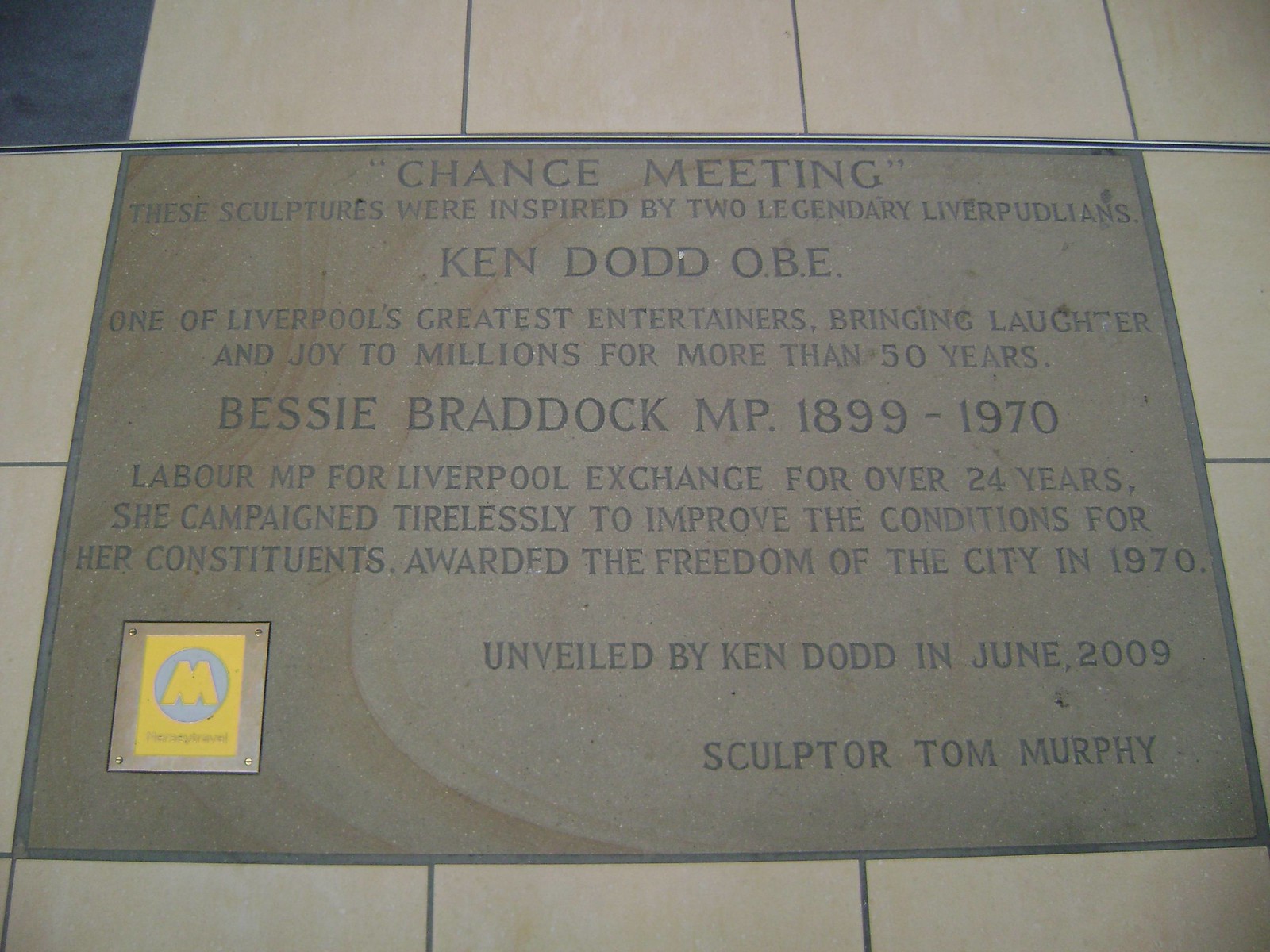The image features an indoor scene showing a gray memorial plaque set into a light-colored floor, presumably made of ivory-colored tiles. The plaque is engraved with a description about sculptures titled "Chance Meeting," inspired by two legendary Liverpudlians. These include Ken Dodd OBE, a renowned entertainer from Liverpool who brought joy to millions for over 50 years, and Bessie Braddock, a Labour MP for Liverpool Exchange from 1899 to 1970, who campaigned tirelessly for her constituents and was awarded the Freedom of the City in 1970. The plaque specifies that it was unveiled by Ken Dodd in June 2009 and created by sculptor Tom Murphy. At the lower left corner of the plaque, there is a smaller yellow rectangle with a white circle inside, containing a yellow "M," which might be the logo of Mercy Travel.